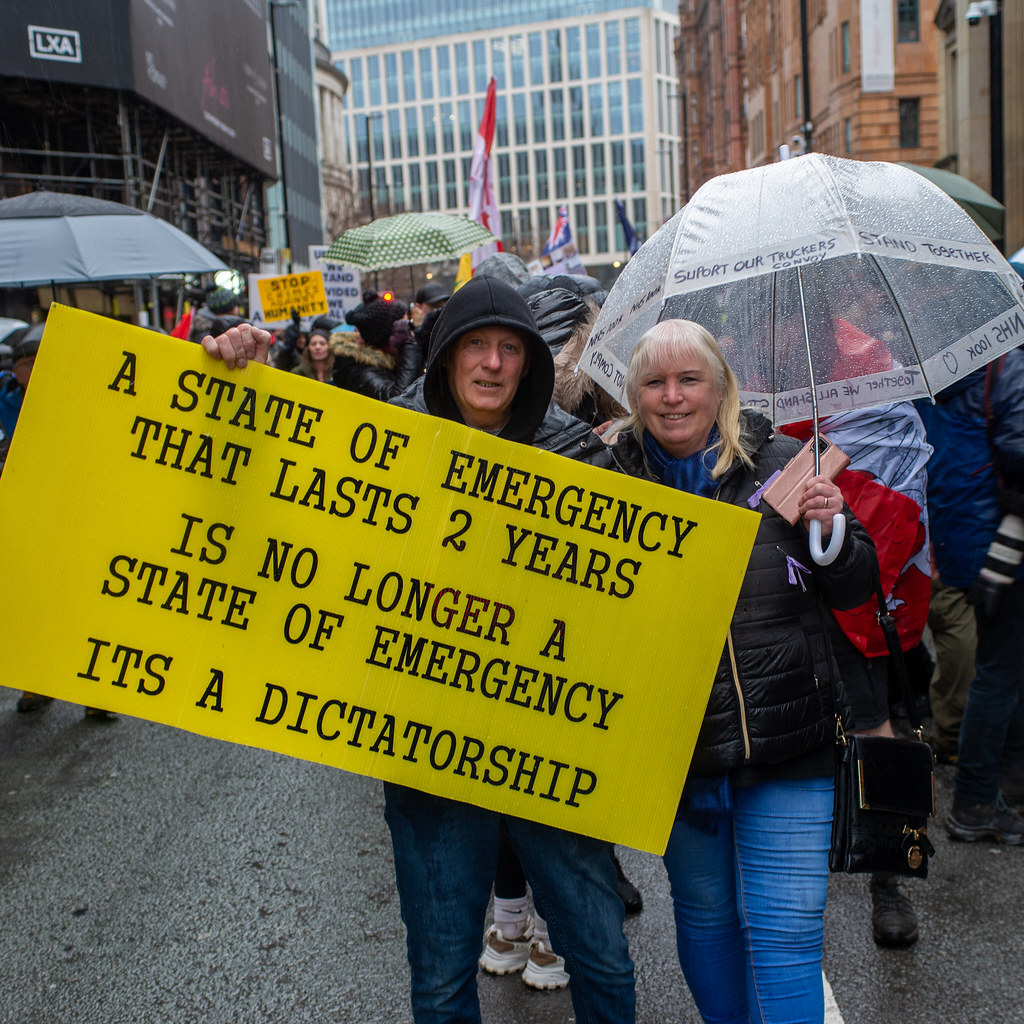In this color, square-format photograph, a dense crowd of people is seen protesting in a downtown area, undeterred by the rain. In the foreground, two individuals stand prominently on a gray asphalt road, facing forward towards the camera. On the left is a man dressed in blue jeans, a black leather coat, and a hoodie with the hood up. He holds a large rectangular yellow sign with bold black text that reads, "A state of emergency that lasts two years is no longer a state of emergency, it's a dictatorship." To his right is a woman with long blonde hair, clad in blue jeans, a black puffy coat with a gold zipper, and a blue scarf. She holds a pink phone, a transparent umbrella with a white handle, and a purse on her arm. The crowd behind them is also equipped with umbrellas of various colors, glistening with raindrops. In the background, metal scaffolding and city high-rises, including a glass building with a beige metal frame and an orange-brown stone building, frame the scene, emphasizing the urban setting. The overall style of the image captures a realistic representation of a moment in a protest, showcasing both the determination of the participants and the dreary weather conditions.